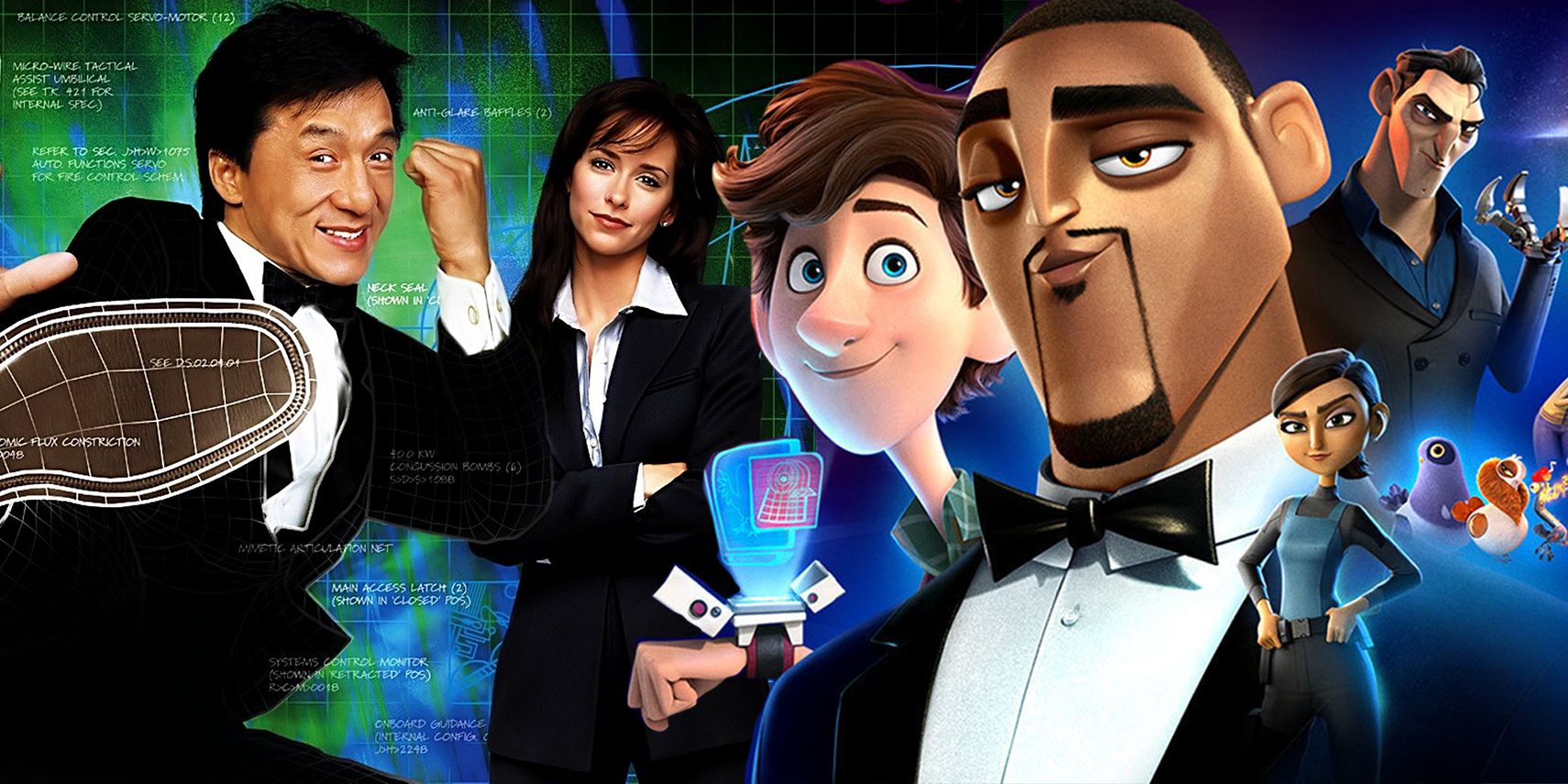This image appears to be a highly detailed and eclectic movie poster featuring both live-action and animated characters, creating a vibrant and intriguing collage. On the left side, renowned action star Jackie Chan is captured mid-kick, clad in a tuxedo with a black shirt and bow tie, reminiscent of his iconic spy films from the early 2000s. Next to him stands a Caucasian woman in a partially unbuttoned, casual business suit, her folded arms and bemused expression adding nuance to the scene.

The right side transitions into animated characters, led by an African-American spy modeled after Will Smith, wearing a black suit and bow tie, echoing his role in a 3D animated film where his character transforms into a pigeon. Accompanying him is a tech-savvy young boy with blue eyes, dressed in a shirt. A menacing villain with pronounced eye shadows, a five o'clock shadow, and a mechanical hand is also depicted, enhancing the poster’s dramatic flair. 

Additional characters include a woman with tied back hair, donning a police uniform complete with a utility belt and sidearm. The background dynamically shifts from greens on the left to blues on the right, amplifying the contrast between the live-action left and the animated right. This vibrant and detailed amalgamation likely aims to capture the eye, invoking the excitement and adventure of spy-themed children's movies.